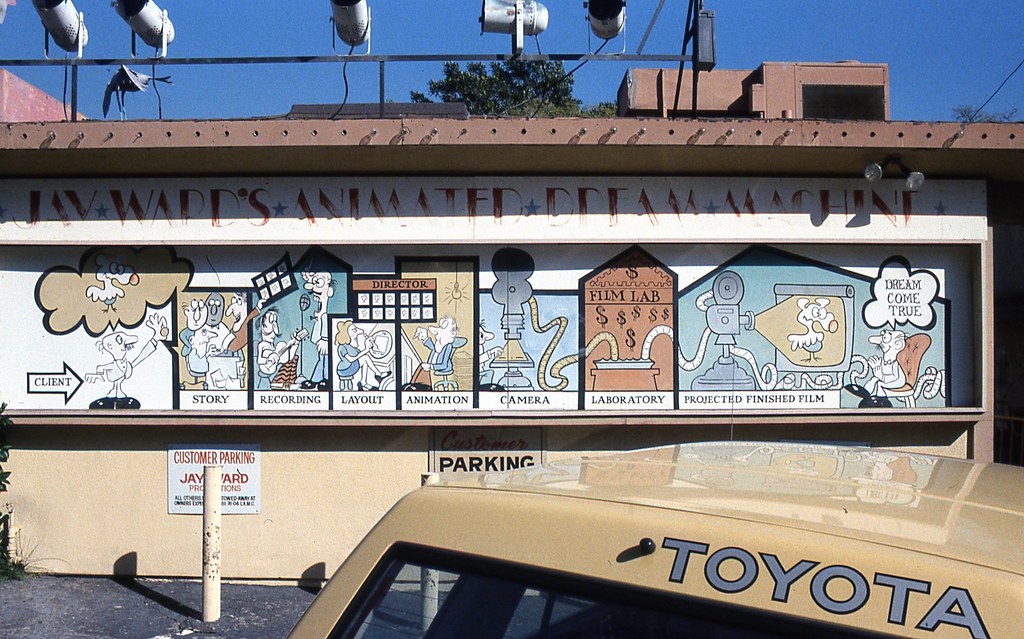This photographic image captures an outdoor scene featuring the facade of a one-story storefront bathed in daylight. Prominently displayed on top of the building is a faded white banner with red lettering that reads "Jay Ward's Animated Dream Machine." Below this banner stretches an extensive mural depicting the steps of animation production.

The mural begins on the left with a cartoon labeled "client," showing a mustached man dreaming about a bird with his hand against a panel. Following this, a panel labeled "story" depicts three men looking over the shoulder of another man who is typing. The next panel, "recording," shows a man playing a guitar while another sings into a microphone. Adjacent to this is the "layout" panel featuring a woman with brown hair, wearing a blue top and skirt, drawing at a desk with the word "director" above her.

Further along, the "animation" panel illustrates a man in a blue jacket sitting in an office chair and waving his hand. After that, the "camera" panel displays a man operating a film camera with film spools. To the right, the "laboratory" panel details the film spools entering a box labeled "film lab" with dollar signs, and concludes with a projector displaying a finished cartoon, proclaiming "projected finished film." The final scene shows the mustached man from the beginning, now smiling and seated in a chair, indicating his dream has come true.

In the foreground of the image is a parking lot featuring tall yellow concrete posts to prevent vehicles from parking too close to the building. There is a gold-colored Toyota parked at the lower right corner of the photo, showcasing its silver logo.

Underneath the mural are the words "Customer Parking Jay Ward Productions Parking," and above the scene, the sky is a clear blue. The brown roof of the building and stage-like lights pointing in various directions add to the detailed composition of this whimsical storefront.